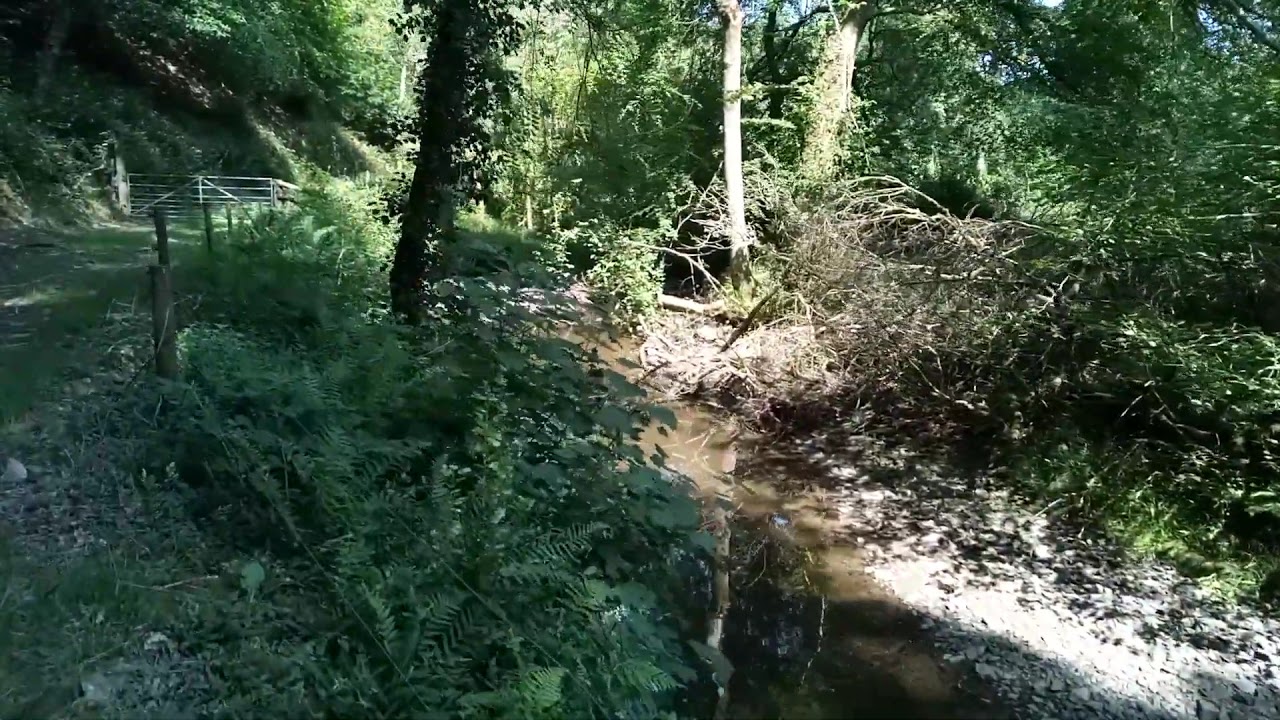The image depicts a grainy photograph of a serene and slightly hilly forest landscape dominated by a creek with brown water running through its center. The creek, which appears more like a small stream or large puddle, is flanked by lush, verdant greenery, including healthy bushes and green branches that stretch out over the water. On the left side, there is a slender tree, while on the right side, white rocks are scattered along the creek's edge. In the background, a metal fence, possibly indicating private property, is visible, with a pathway leading up to it. The scene is characterized by pockets of sunlight filtering through the canopy, creating a contrast with the shadowy forest areas. The setting suggests a tranquil, natural environment suitable for hiking, with abundant trees, dirt, grass, and a mix of living and dead branches, all contributing to a picturesque day in the forest.